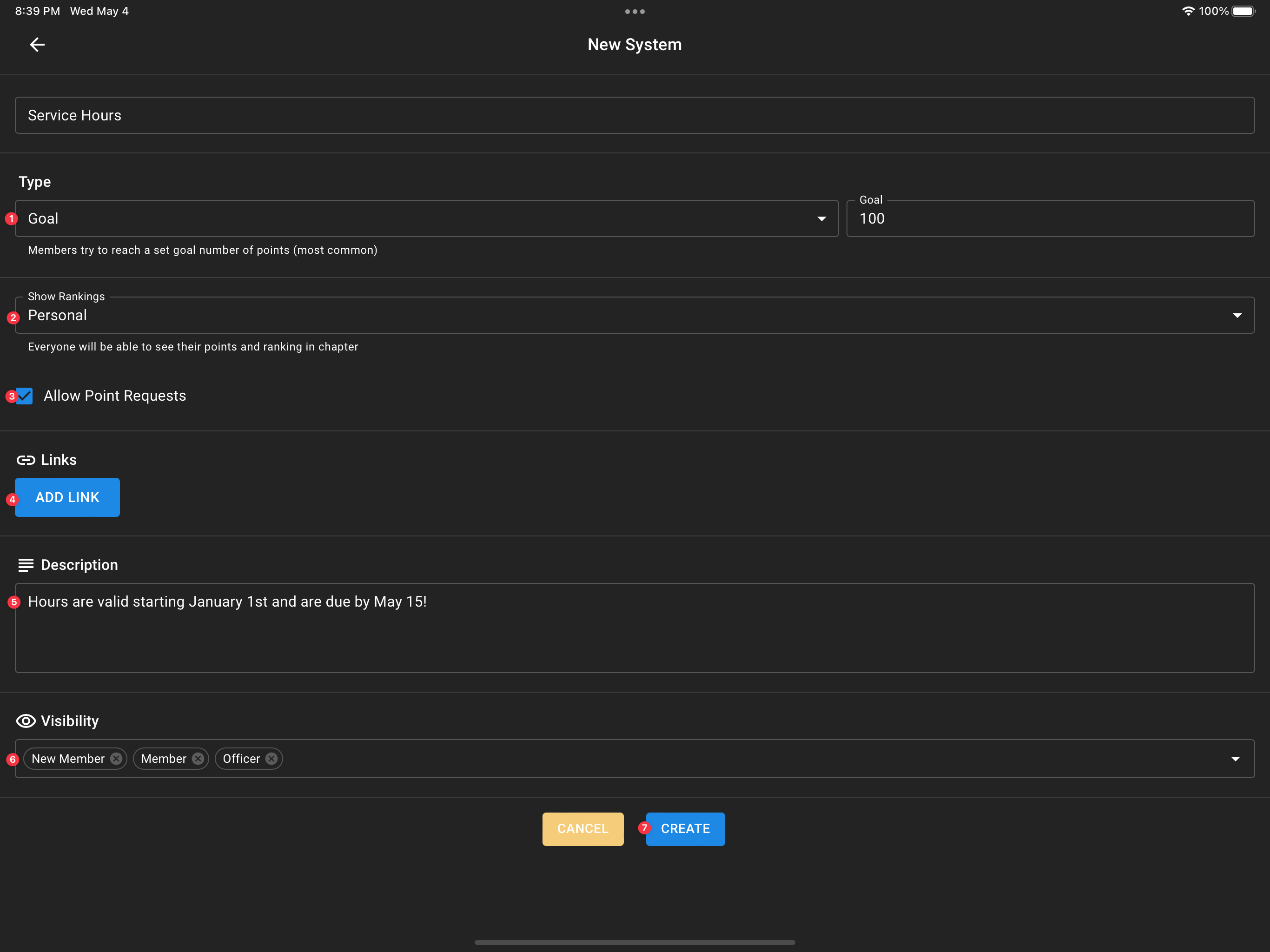In the upper left corner, the time is displayed as 6:39 PM on Wednesday, May 2nd. To the right of the time, indicators show a new system notification and a fully charged phone battery at 100%. 

Below this, an open rectangle labeled "Service Hours" appears. Underneath it, the word "Type" is written, followed by a small red circle beside the word "Goal." Here, members aim to achieve a predefined point target. There is a dropdown option under "Goal" that allows users to select different goals. It indicates "Goal 100" next to it. 

Further down, "Rankings" is listed with the word "Personal" next to another red circle. This denotes that everyone can view their individual posts and rankings. Below this, an option to allow point requests is presented with a checkbox. 

"Links" is mentioned next, followed by a clickable blue rectangle labeled "Add Link." 

A description mentions: "Hours are valid starting January 1st and are due by May 15th." Finally, at the bottom of the section, there are two buttons—one labeled "Cancel" and the other labeled "Create."